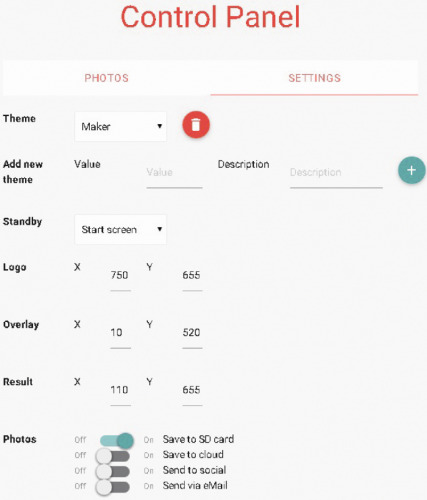The image showcases a control panel page with various settings and options. At the top of the page, the heading "Control Panel" is prominently displayed in orange text. Beneath this are two tabs labeled "Photo" and "Settings," also in orange. The "Settings" tab is highlighted and underlined in orange, indicating it is the active selection.

On the left side of the page, there are several options under the "Settings" tab. The first option listed is "Theme," with "Maker" selected from a dropdown menu. Below this is an orange "Delete" button. Additional settings include fields labeled "New Theme," "Value," and "Description." Further down, there is another dropdown menu for "Standby," which currently displays "Start Screen."

Coordinates for various elements are also displayed:
- Local X: 750, Local Y: 655
- Overlay X: 10, Overlay Y: 520
- Result X: 110, Result Y: 655

At the bottom of the page, there is a section labeled "Photos," displayed in orange text. This section contains four toggle switch settings:
1. "Save to SD Card" – the switch is on and blue.
2. "Save to Cloud" – the switch is off and gray.
3. "Send to Social" – the switch is off and gray.
4. "Send via Email" – the switch is off and gray.

The background of the image is a light gray shade, and the majority of the text is black, creating a clear contrast for easy readability.